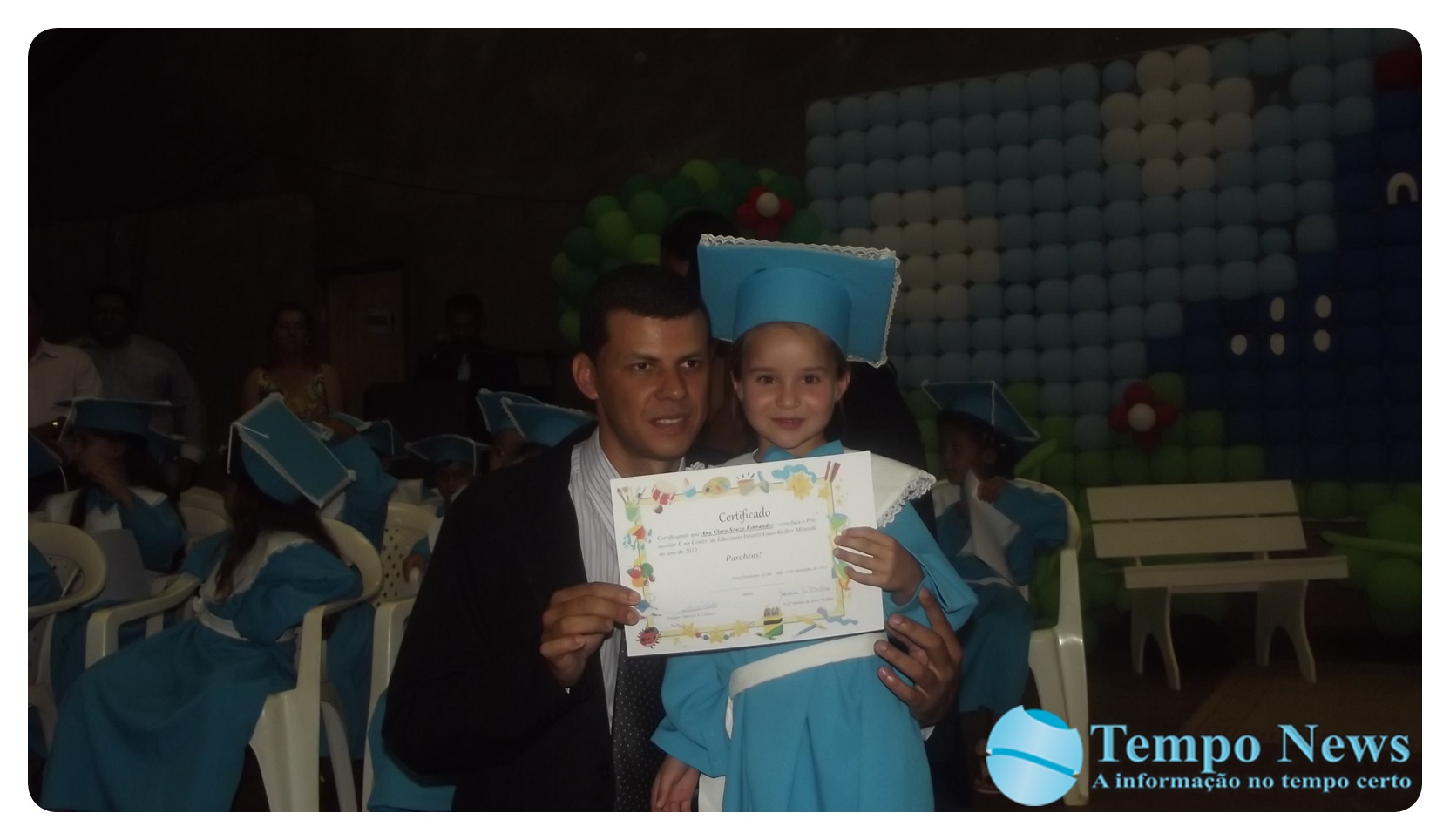This is a full-color, yet very dark photograph capturing a tender moment at a kindergarten graduation event. Front and center, a father kneels beside his young child, who is dressed in a blue graduation gown and mortar board. The father, who has dark hair and is wearing a white striped shirt beneath a dark blue or black jacket, helps hold up a colorful certificate, likely the child's diploma. To the left, other children in similar blue gowns and mortar boards can be seen seated in the background. A wooden bench is visible to the right. Written in light blue text is "Tempo News," suggesting the source of the image. The setting appears to be indoors at a school or academy, with limited lighting adding to the intimate atmosphere of the celebration.